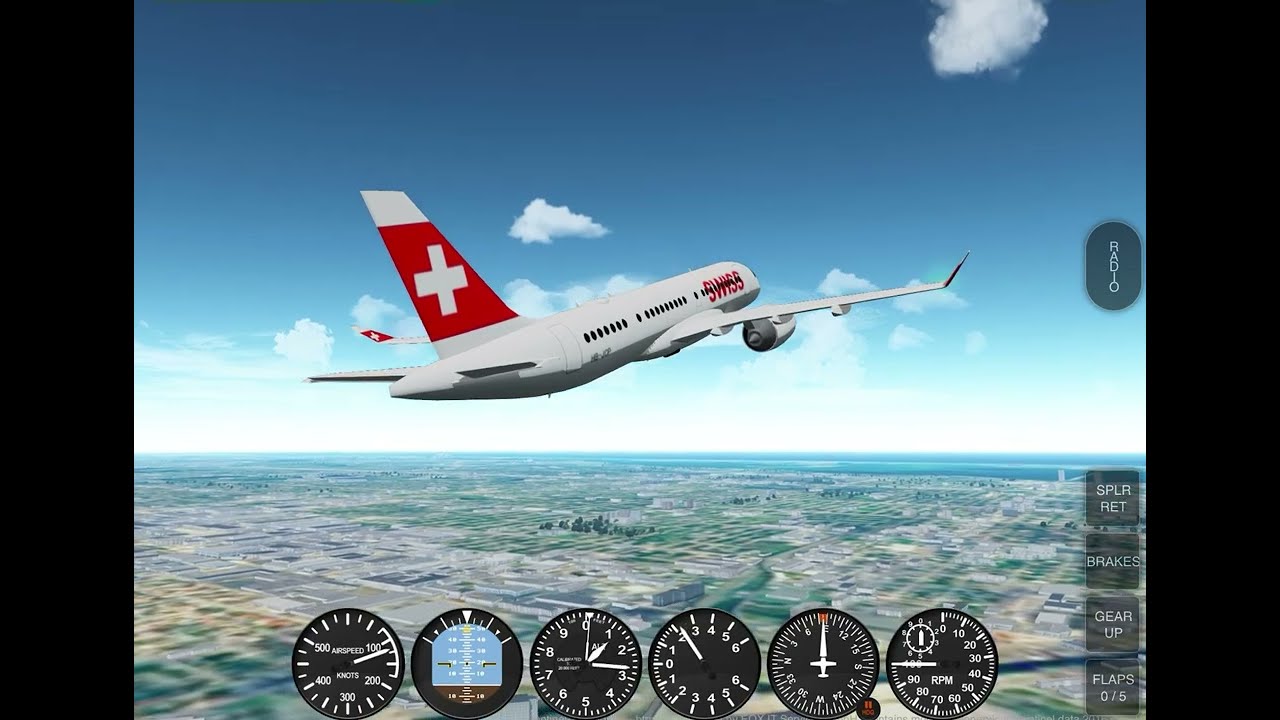This image is a detailed screenshot of a video game airplane flying through the sky, angled to the right and away from the camera. The airplane, prominently white with red accents, has the word "Swiss" written in red on its front body, and a red tail with a distinctive white cross. The blue sky, dotted with a few puffy white clouds, forms the background, while below, you can see green terrain, parcels of land, various trees, and the blurry silhouettes of buildings, indicating the plane is relatively low to the ground. Streets are visible amidst the landscape. At the bottom of the image, six black circular gauges display information such as speed, altitude, and direction, similar to those found in a car's dashboard.